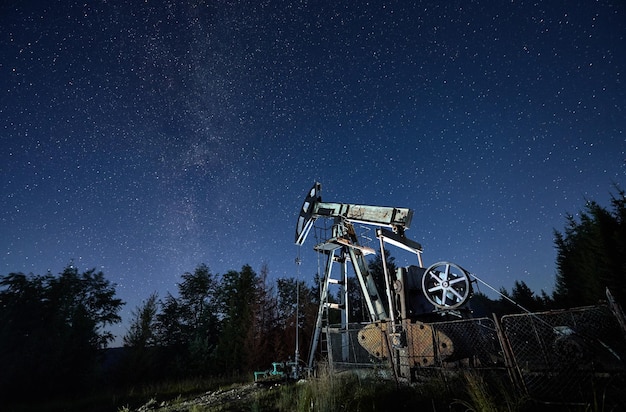The image depicts an old, rusted oil rig set atop a small hill, surrounded by tall pine trees that seem to reach into the night sky. Enclosed by a worn, broken-down fence, the oil rig stands silently, appearing unused and stationary. Below, some plants sprout from the ground, adding to the remote and desolate atmosphere. The night sky above is a deep navy blue, illuminated by hundreds of tiny specks of light—stars and other celestial entities—which gradually grow denser as the night deepens. A solitary light on the rig highlights its machinery, contrasting it against the expansive, star-lit background.